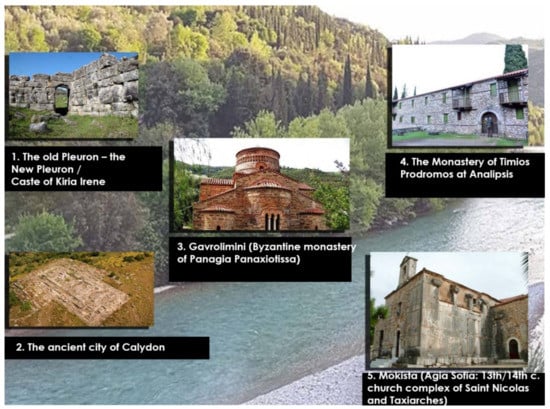The background of the image is a picturesque view of a river meandering through a verdant ravine. The left bank of the river is lined with a variety of foliage, including green bushes, towering pine trees, and other diverse plant life, some of which appear dried or yellowed, adding an autumnal touch to the scene. The river itself is notably broad, displaying a vibrant blue-teal hue as it flows. On the right side of the river, a rugged rocky coast can be partially discerned.

Over this natural setting, five smaller images have been strategically placed, forming an informative collage:

1. **Top Left Image**: This image depicts ancient ruins. Below it, within a black box, white text reads: "The old Pluron, the new Pluron castle of Curia Irene."
2. **Below the First Image**: A photograph of a field is presented. Accompanying text in a black box beneath the image states: "To the ancient city of Caledon."
3. **Center Image**: Placed prominently, this image features a temple-like structure. The caption within a black box reads: "3 Gavrilmini Byzantine Monastery of Panagia Panagialissa."
4. **Top Right Image**: This image shows an elongated building. The description, displayed in a black box with white text, says: "For the Monastery of Timios Prodromos of Annapolis."
5. **Below the Fourth Image**: The final image in this collage appears to be of a larger church. The black box beneath it describes: "5 Mochista Agios Sophia 13th-14th Century Church Complex of St. Nicholas and Taxiarches."

This detailed caption endeavors to capture the essence and information conveyed by the composite image.